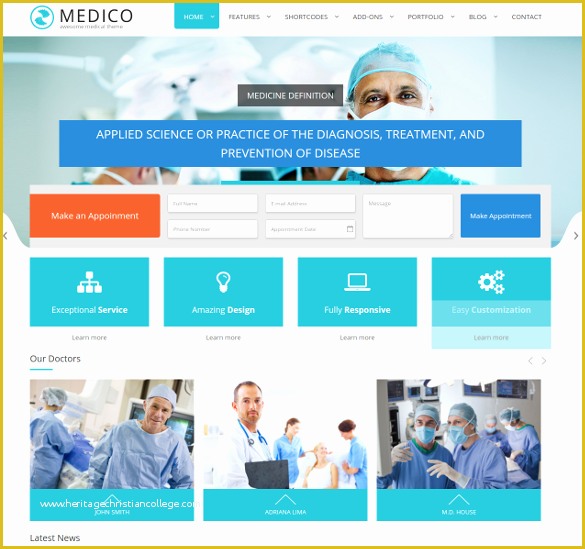The image features a predominantly white background with a busy layout. A mustard-colored border frames the top left corner, where a circular logo with a 'Z' is situated, accompanied by the black text "Medico, Medico." Below this, a series of navigation tabs are aligned in a horizontal row. The first tab, in teal with white text, reads "Home," while the other tabs in black cover various categories: "Features," "Shortcodes," "Add-ons," "Portfolio," and "Blog Content."

A prominent visual element is an image of a health professional adorned with a teal hairnet and a white mask. Partially overlaying this image is a blue rectangle with a white inscription that reads, "Apply science or practice of the diagnosis, treatment, and prevention of disease." Above this blue rectangle, a black rectangle features the white text "Medicine Definition." Below, on the left-hand side, a conspicuous orange box contains the text "Make Appointment" in white.

The lower section includes several teal boxes with white text detailing different features: "Exceptional Service," "Amazing Design," "Fully Responsive," and "Easy Customization." Additional content features images of health professionals alongside what appear to be names, including "Adriana Lima, MD," possibly indicating their expertise or roles.